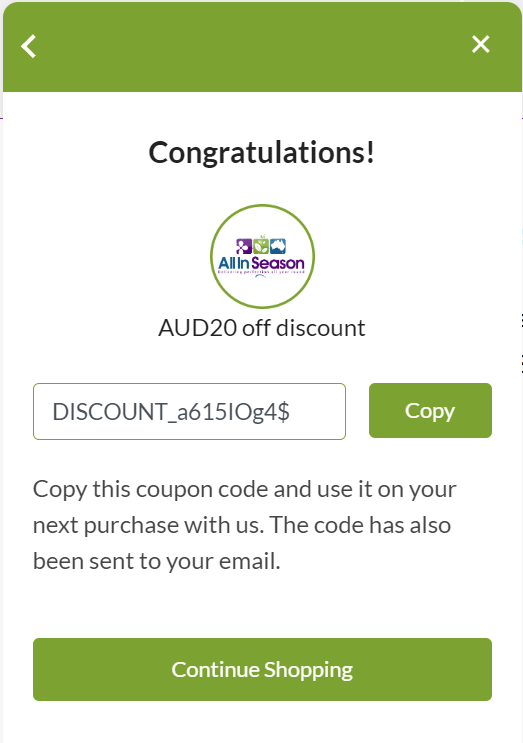This image depicts a pop-up window layered over another window. In the upper border of the pop-up, there is a small white "X" located at the top right corner, indicating the option to close the window. The background behind this pop-up appears to be gray with some black lines, suggesting underlying text.

The pop-up itself has a muted green border at the top, featuring a white back arrow on the left and a close icon (white "X") on the right. On a white background within the pop-up, bold black text announces, "Congratulations!" Below this, there is a green circular border around a white circle containing the text, "All in Season."

Following this, it advertises an AUD $20 off discount with a coupon code. The discount code is displayed in a green rectangular box with black font: "Discount_A615IOG4$". A green button with white text that reads "Copy" is positioned adjacent to the code.

At the bottom, instructions in black font direct the user to "Copy this coupon code and use it on your next purchase with us. The code has also been sent to your email." The pop-up concludes with a green button, also in white font, prompting the user to "Continue shopping."